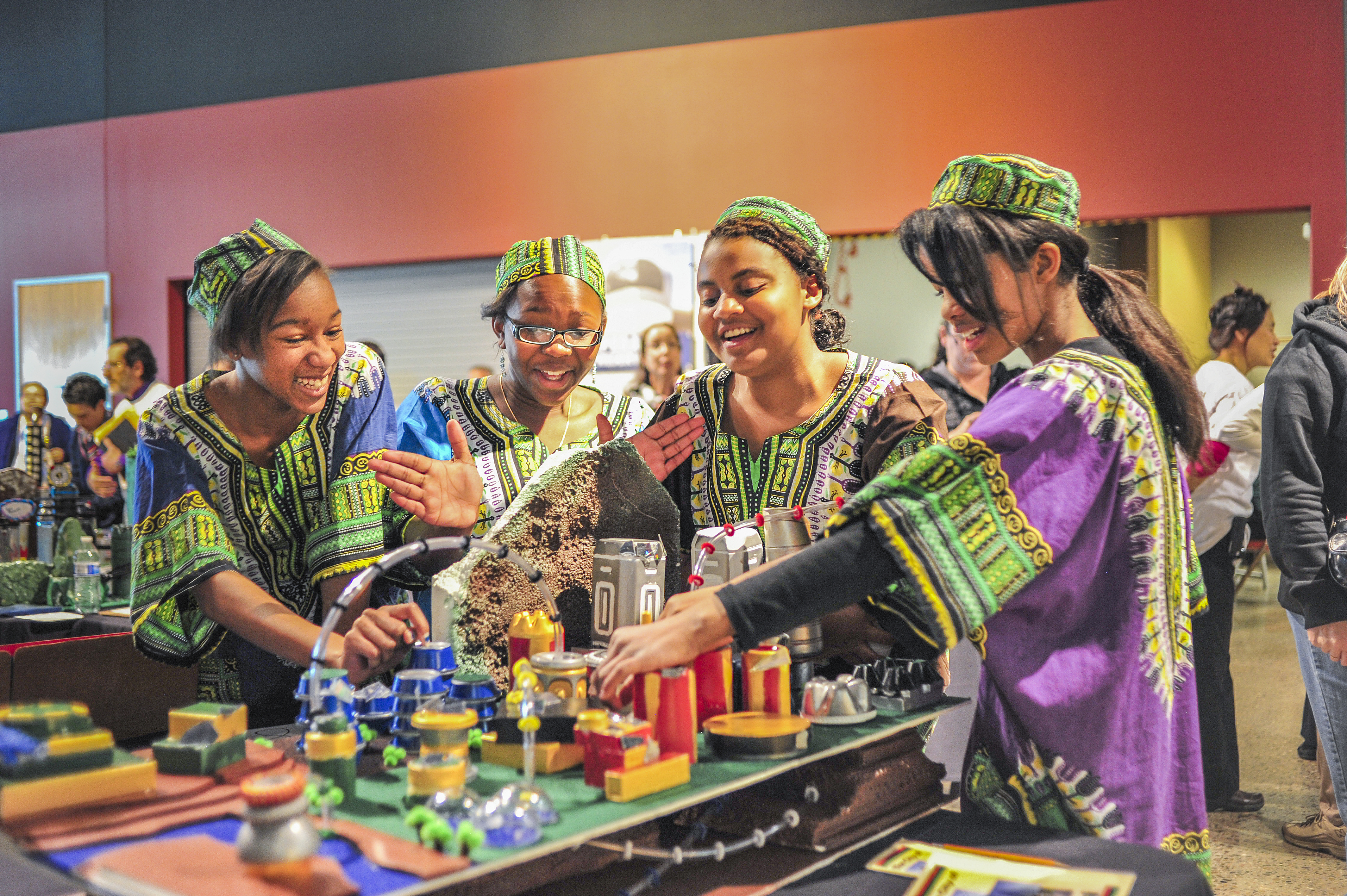The photograph captures an indoor exhibition scene with vibrant details and cultural elements. At the forefront, four girls, all dressed in traditional African attire, are gathered around an intricate model displayed on a table. The model appears to represent a cityscape or similar landscape, complete with various objects attached to it, including tubes adorned with red and black ties. The base of the model is green, simulating grass, and includes features that replicate water.

In the background, the exhibition area, which has red walls transitioning to black towards the top, is bustling with other visitors in western attire, either standing or moving around the space. The striking colors and cultural differences between the participants and the observers add depth and contrast to the scene.